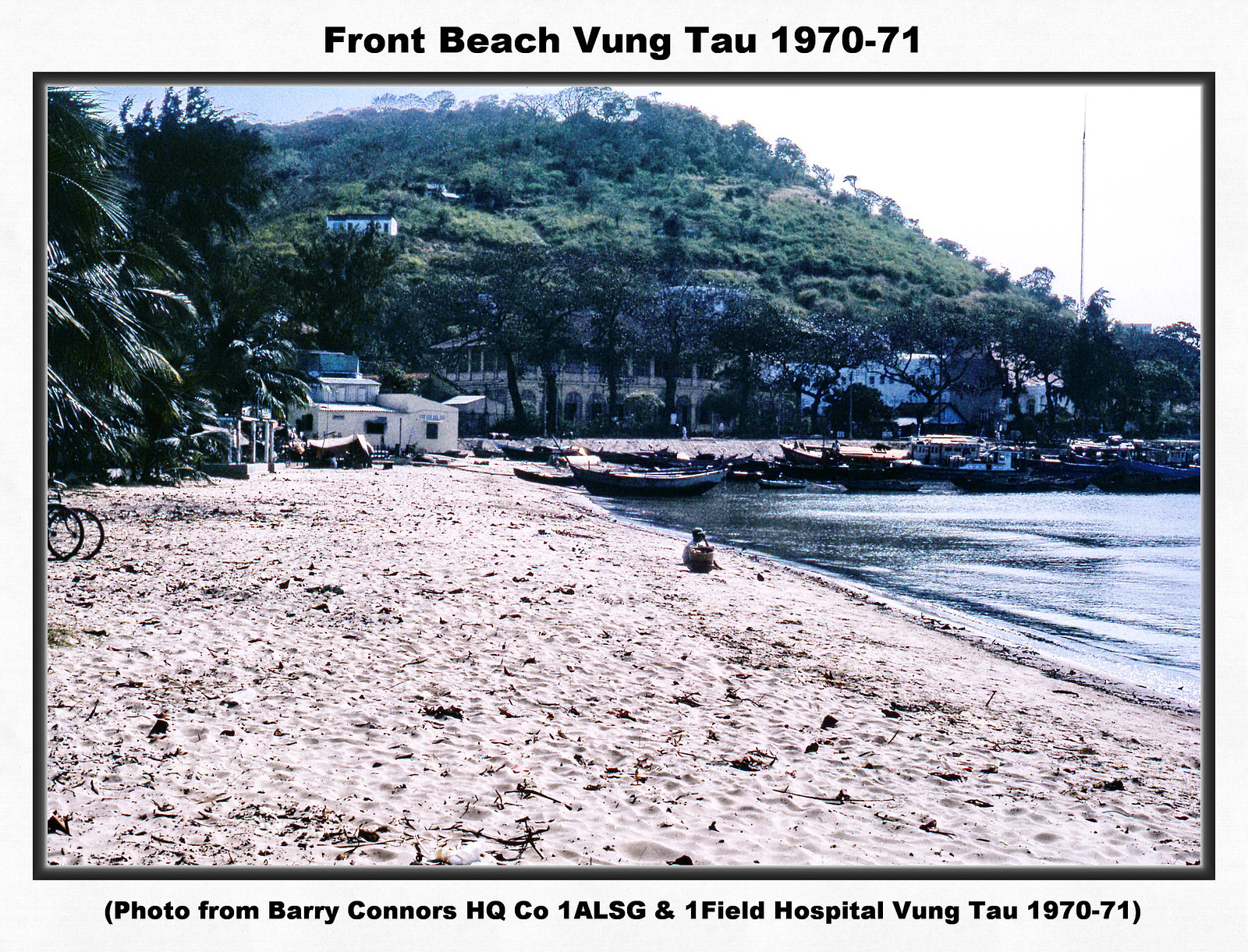This detailed color photograph, bordered in black and featuring a gray band at the top, depicts Front Beach, Vũng Tàu, during the years 1970-71. An inscription above reads "Front Beach VŨNG TÀU 1970-71," while a note at the bottom states, "Photo from Barry Connors, HQ CO 1A LSG N1 Field Hospital, VŨNG TÀU, 1970-71." In the image, a serene beach stretches along the foreground, leading towards moored boats that extend from the center to the right edge of the frame. Beyond the boats, additional stretches of the beach are visible, with white buildings lined up further back, seamlessly blending into lush, bush-covered hills that form a mountainous backdrop. On the left side of the beach, occasional trees punctuate the scenery. A single figure, possibly squatting with a basket nearby, can be seen just right of center, adding a human element to the tranquil scene.